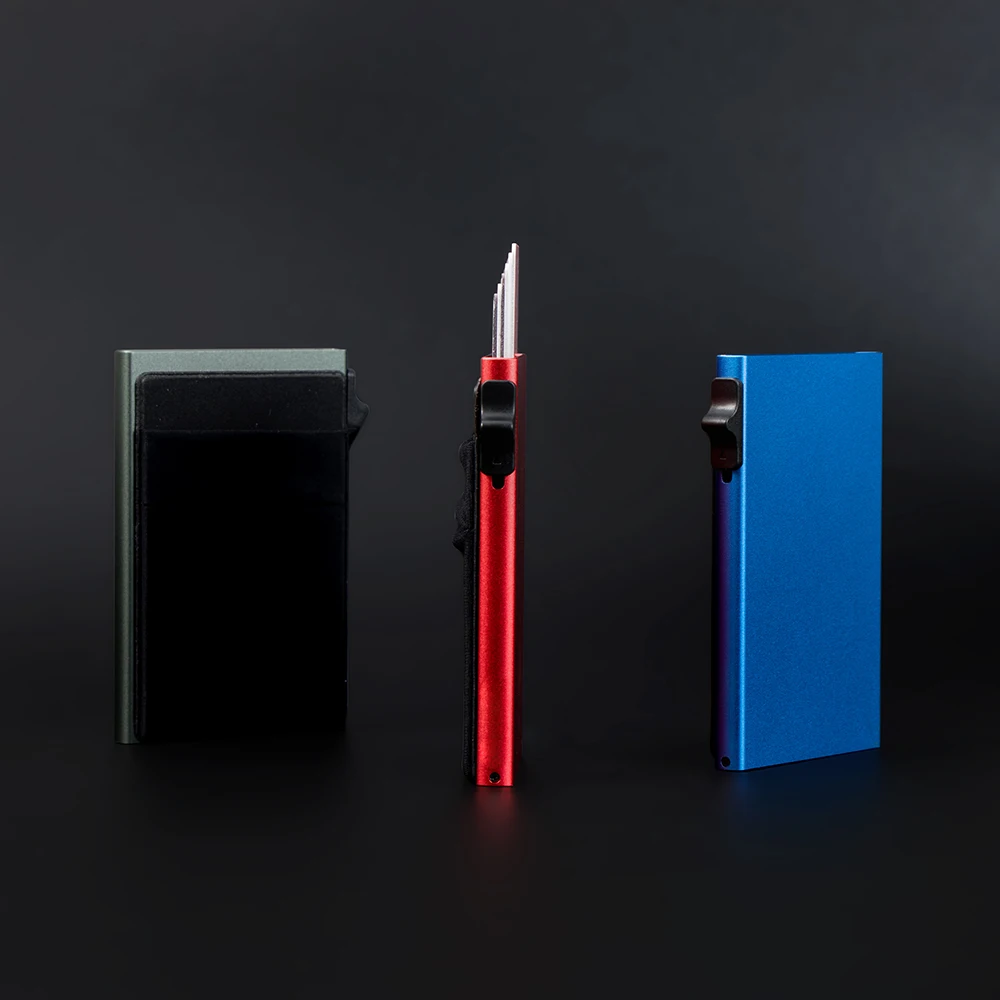The product photograph showcases three sleek and modern card holders, each floating seamlessly in a dark gray void. This sophisticated editing style, featuring a solid dark gray surface and background, is typically used for commercial settings such as online shops, websites, or catalogs. On the left, the card holder displays a black outer case encasing a silver interior, with a black knob on the right side. The middle card holder is shown in a side profile, emphasizing the black knob and a fanned arrangement of multiple cards, clearly indicating its function as a business card holder. The rightmost card holder stands out with its vibrant blue color, completing the trio. The stark, minimalist presentation highlights the product's functionality and elegant design, ideal for professional use.